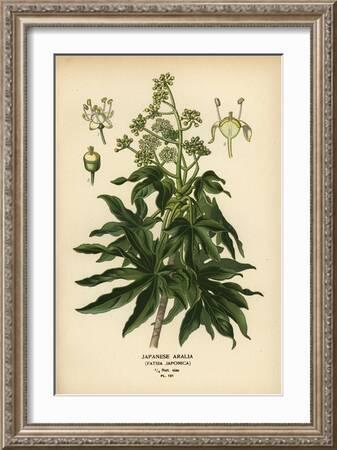The image depicts a detailed botanical illustration of the Japanese Aralia plant, characterized by a series of broad, green leaves branching out from a thin, light brown or grayish stem. The plant also features clusters of tiny buds at the top that resemble dill flowers. The artwork is presented against a light peach or apricot background, creating a soft contrast with the white border surrounding it. This border is encased in an ornate, multi-layered picture frame that appears to be light brown or perhaps an intricate silver-gold finish. Below the central illustration, the caption "Japanese Aurelia" is prominently displayed, followed by three additional lines of smaller, unreadable black text. The overall composition of the image suggests a scientific or botanical reference, emphasizing the plant's distinct features.